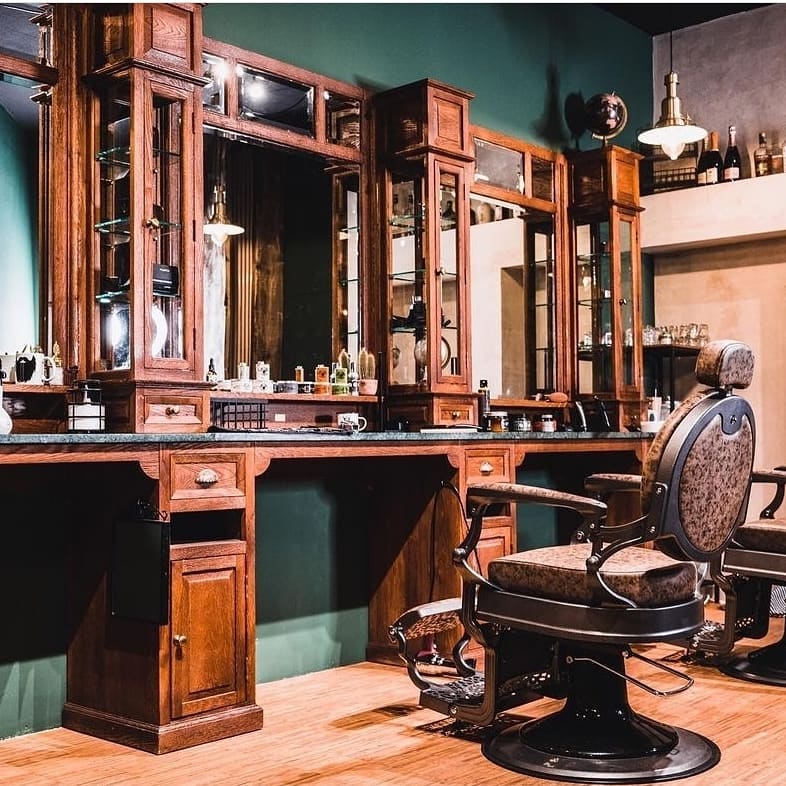The image depicts a meticulously detailed, vintage-style barbershop that makes one wonder if it is a modern recreation or an AI-generated scene. Central to the left is a wooden barber stand, adorned with a bluish-green countertop, holding various ointments, styling gels, and other barber tools. The countertop is set in front of windows, facing where a customer would sit. The barbershop features wooden and glass cabinetry, complete with mirrors between pillars, and a granite countertop. A white wall at the back hosts a chandelier and a row of wine bottles on top, alongside a globe on one of the pillars in the corner. The prominent barber chairs, suggestive of the 1950s-1960s era, are highly stylized with metal bases, armrests, cushions, and footrests; one is partially cut off in the image. The flooring is wooden, and the wall behind the cabinets is a darker green with a lighter green base trim, contributing to the vintage aesthetic. Additionally, other walls display a beige tone, with hanging lights adding to the ambiance. Several objects—brushes, glasses, and possibly hair-cutting or shaving tools—are scattered across the area, completing the rich, nostalgic scene.